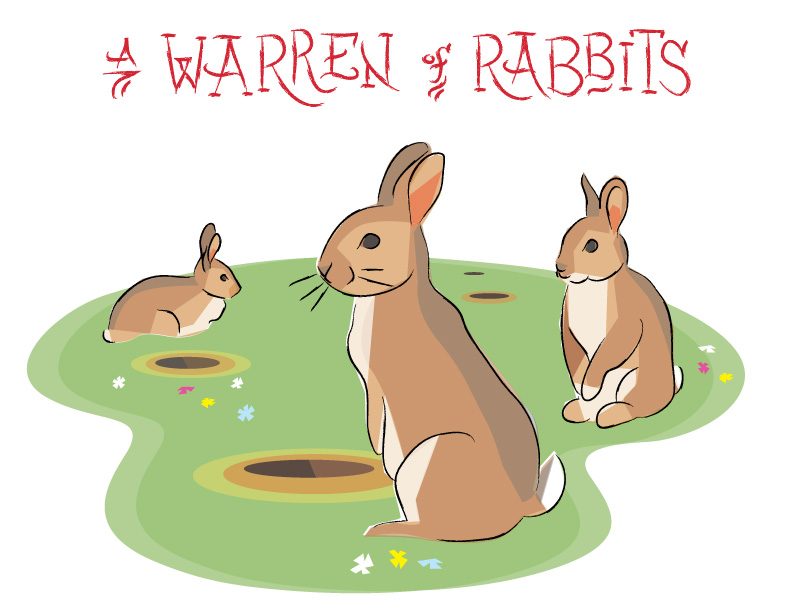The image is a whimsical, hand-drawn illustration suited for a children's book cover titled "A Warren of Rabbits," written in playful, pencil-like red text at the top. Set against a stark white background, the scene features three brown rabbits with white cottontails and cream-colored bellies, positioned around an irregularly shaped, light green patch of grass adorned with tiny, stylized flowers in pink, yellow, white, and blue. The rabbits are depicted with a cartoonish flair: one lies down on the left, another sits upright on its haunches at the forefront looking left, and the third, slightly smaller, sits at a slight angle to the right behind the second rabbit. Scattered across the grassy area are three to four drawn rabbit holes, adding a playful, detailed touch to the scene. The overall simplicity of the design, combined with the creative text, gives the image a charming, childlike appeal.